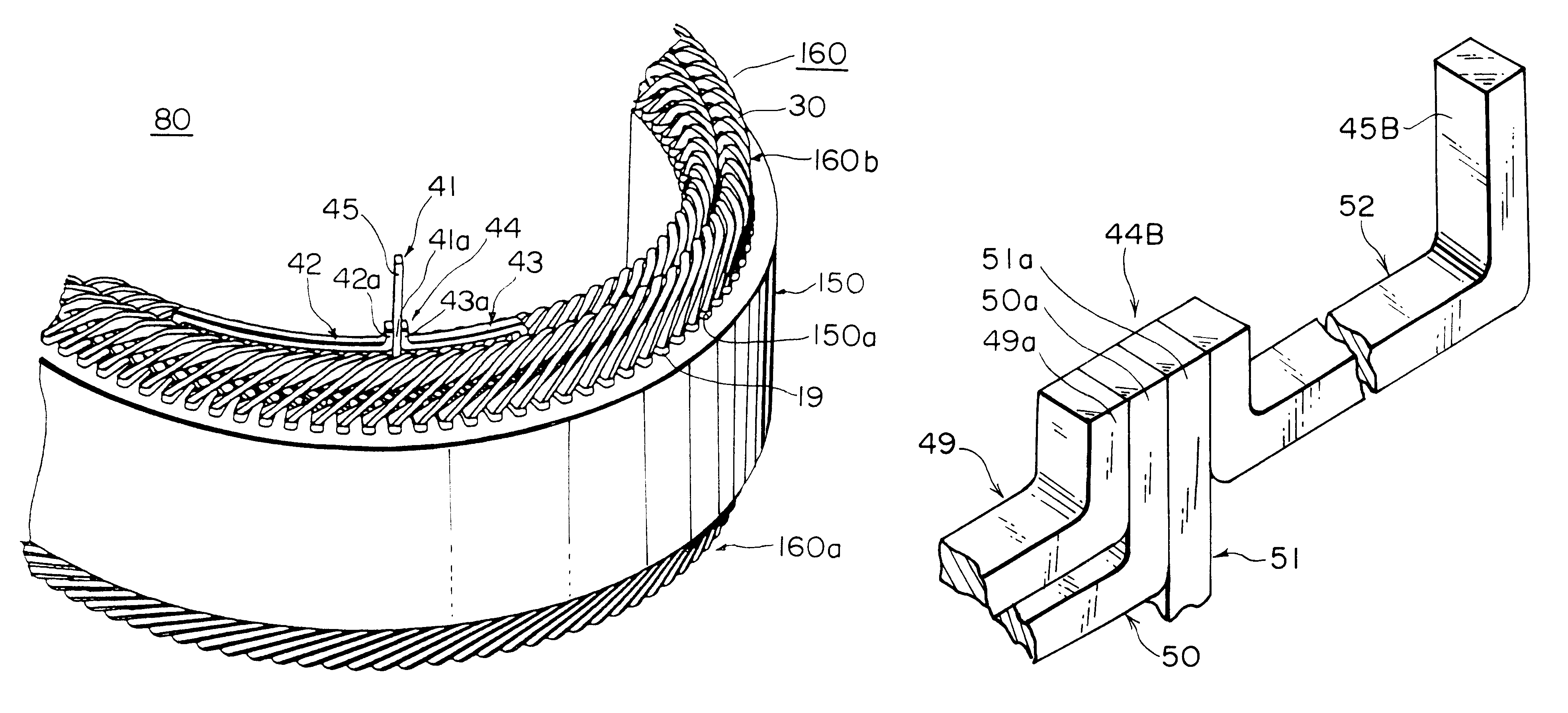The image showcases a detailed black-and-white blueprint of two adjacent structures. The structure on the left is curved and resembles a semi-circular or diaphragm shape, featuring sharp, layered components on top and a vertical rod extending upwards. This structure is meticulously labeled, with parts marked by numbers such as 80, 41, 41A, 42A, 42, 43, 43A, 44, 45, 160, 130, 160B, 150, 150A, 19, and 160A. The diagram is set against a plain white background and includes several lines pointing from these labels to specific parts of the structure.

To the right, there is another uniquely shaped structure, resembling a backward L attached to a long U or a cylindrical, rectangular piece assembled from multiple components. This structure is also labeled with various numbers and letters, including a notable underlined number 80 at the top left. The detailed lines and numeric labels suggest that the diagram may be part of a patent or a technical drawing, possibly related to a steam engine or turbine device. The overall presentation suggests a highly detailed and technical blueprint, aimed at providing a thorough understanding of the device's components and assembly.